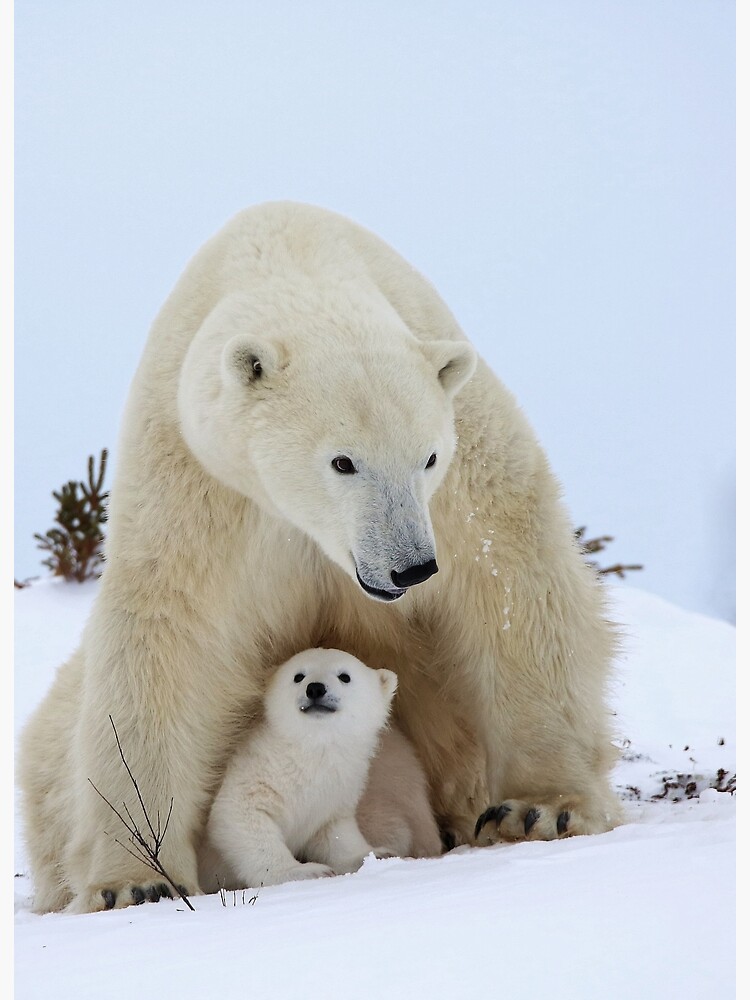In this captivating nature photograph, a protective mother polar bear and her cub dominate the scene, showcasing the tender bond between them. The foreground presents a diagonal slope covered in pristine, white snow, with a small black stick poking through on the left side. The mother polar bear, large and imposing, has cream-colored fur with a slightly whiter head. Her black nose, eyes, and small ears stand in stark contrast, while her body forms a triangular shape as she hunches over her cub. Her long, black claws grip the snowy surface. The cub, significantly smaller and whiter, nestles between her feet near her belly, facing forward. Their sharp black features – eyes, nose, mouth – mirror each other. The background consists of a light blue and gray sky, with sparse dark green bushes dotting the snow-covered landscape, adding a hint of rugged terrain to this cold, serene habitat.